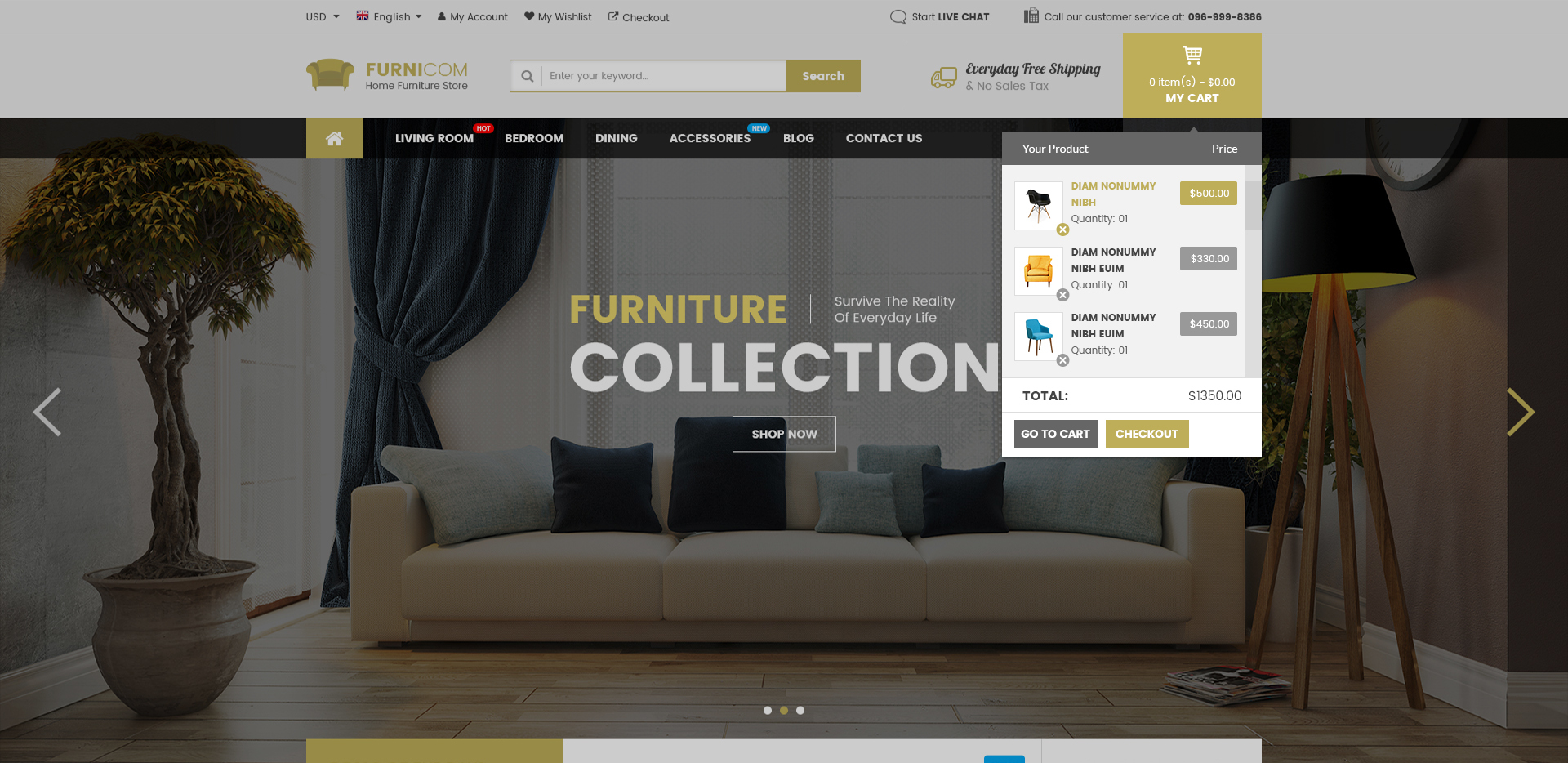Screenshot of a furniture e-commerce website, Ferny.com. The top left corner features a navigation bar with options such as USD currency, English language settings, "My Account," "My Wish List," and "Checkout." On the top right, a speech bubble icon labeled "Start Live Chat" is displayed, alongside a customer service number. Below, a search bar is situated next to a "Search" button. To the right, the phrase "Everyday Free Shipping" is highlighted with a yellow truck icon. Adjacent to this, a yellow shopping cart icon indicates zero items and a zero-dollar total. 

Progressing down, there's a primary navigation menu within a black bar, showcasing links to "Home," "Living Room," "Bedroom," "Dining," "Accessory," "Blogs," and "Contact Us." Just beneath this menu, a prominent image of a beige sofa is displayed, adorned with three main cushions and multiple decorative gray and black pillows. To the left, a potted tree in a stone vase and large blue curtains frame expansive windows in the background. On the right, a unique lamp with a triangular four-legged base and a black lampshade emits a soft yellow light. Navigation arrows on either side of the sofa image hint at further browsing options.